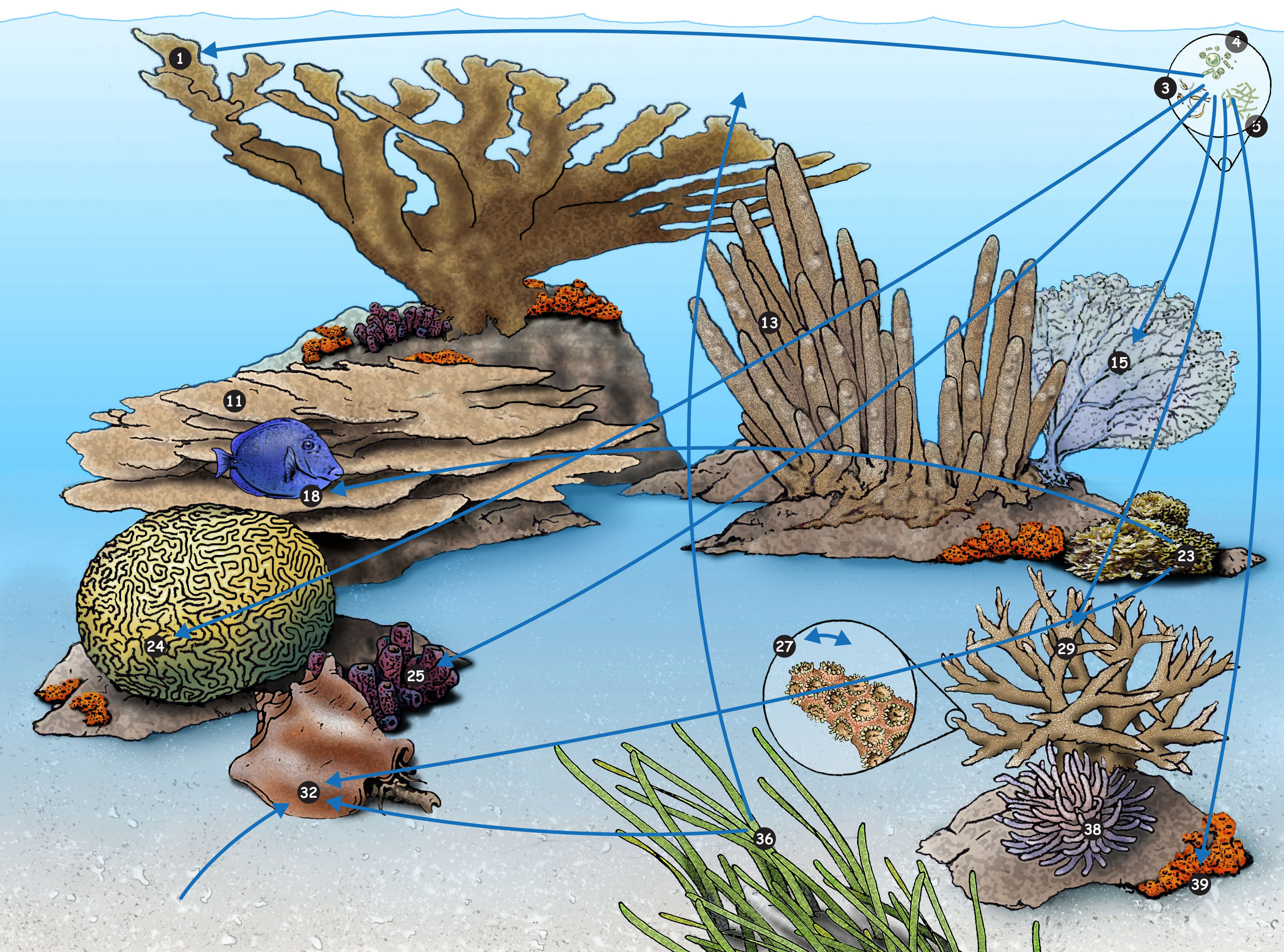The image is a detailed underwater illustration showcasing an array of vibrant corals, marine plants, and sea creatures, each meticulously labeled with numbers. Prominently, a blue fish marked with the number 18 swims among the formations. The diverse collection of corals includes a brain coral numbered 24, purple tube-like corals numbered 25, and various others sequentially numbered. A significant conch shell stands out, labeled 32, alongside seagrass marked 36. In the top right corner, there's a circle containing microscopic organisms or plankton numbered 3, 4, and 5, with blue arrows extending from these to different parts of the coral, indicating relationships or dependencies. Key elements also include a green sponge-like creature labeled 23, a fan-like gray structure numbered 15, and an anemone-like organism numbered 39. Additional elements such as a tan, leaf-like creature marked 11 and various other uniquely described and numbered sea flora and fauna fill the scene, painting a comprehensive picture of underwater biodiversity.